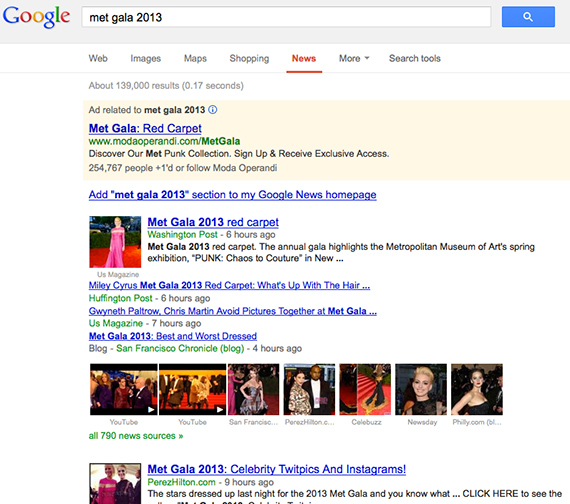In this screenshot of a Google search results page, the top left features the iconic Google logo. To its right is the search box where the query "Met Gala 2013" is entered. Adjacent to the search box on the far right is the blue search button. 

Beneath the search bar, there are various tabs for filtering results, including "Web," "Images," "Maps," "Shopping," "News," "More," and "Search Tools." In this instance, the "News" tab is selected, indicating a specific search for news articles.

The search results indicate "about 139,000 results in 0.17 seconds." At the top of the results, there is a beige-highlighted ad related to the Met Gala 2013, featuring a clickable information icon. The ad links to a website titled "Met Gala Red Carpet" at modaoprandi.com/MetGala.

Further down, there is an option to add a "Met Gala 2013" section to the Google News homepage. Following are news articles from various sources including The Washington Post, The Huffington Post, U.S. Magazine, and the San Francisco Chronicle blog. Each of these articles discusses different aspects of the Met Gala 2013. Additionally, there are related images including YouTube video thumbnails, with the final source being PerezHilton.com.

This detailed caption provides a comprehensive overview of the search results and layout for the query "Met Gala 2013."